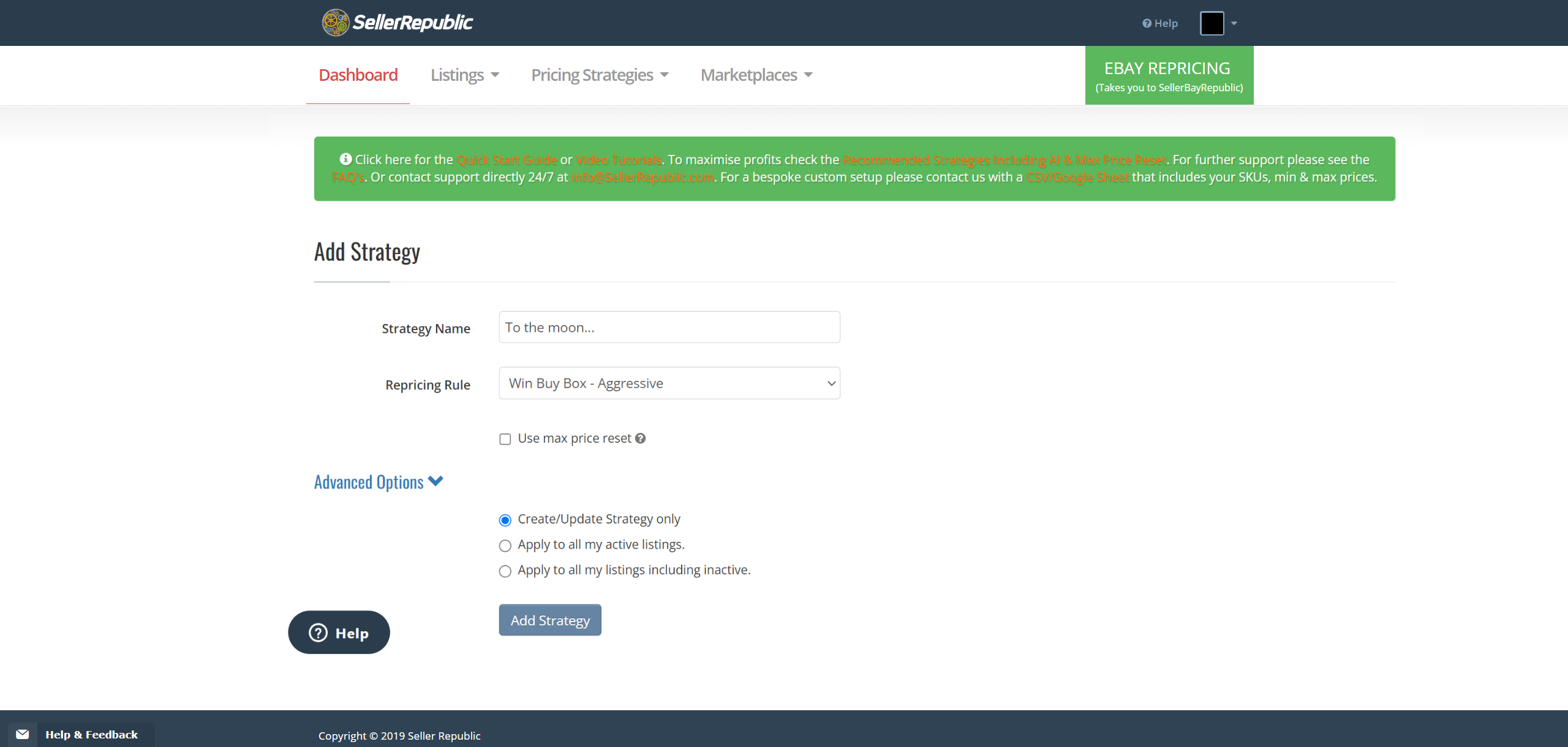The image depicts the dashboard of the SellerRepublic website. The dashboard is the current section displayed, with other options such as Listings, Pricing Strategies, and Marketplace available for selection. Within the dashboard, users can develop and name specific pricing strategies, select repricing rules, set maximum prices, and configure a variety of advanced options. Once configured, users can finalize their strategy by clicking the "Add Strategy" button.

SellerRepublic appears to function similarly to eBay, where users can list items for sale and create bulk listing strategies to streamline their selling process. An interactive help feature is available in the bottom left corner, signified by a "Help" button accompanied by a question mark icon. Additionally, a help and feedback email address is provided in a banner at the very bottom of the screen, which also contains a copyright notice indicating the site was established in 2019. This implies that SellerRepublic is a relatively new platform, having been in operation for approximately five years.